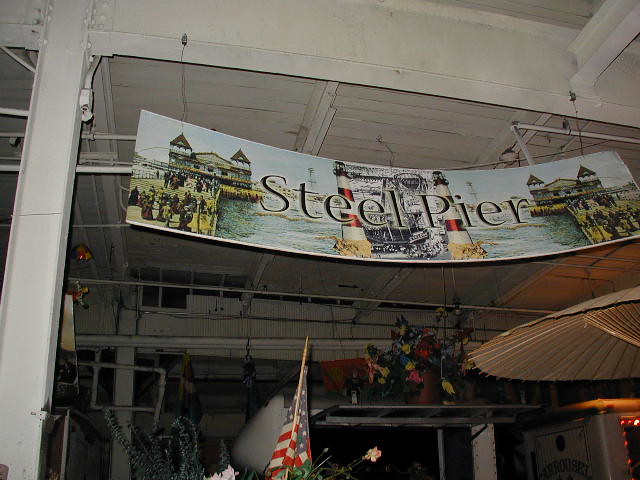The image captures an intricate and aged painting on a hanging banner that reads "STEEL PIER" in large letters across the center. Set in a warehouse-like room with gray wooden slat ceilings and metal beams, the banner showcases a detailed coastal scene. The painting depicts multiple lighthouses—one on the left, one in the center, and one on the right. These lighthouses are characterized by their distinct red and white colors. Below each lighthouse, there are buildings jetting out into a blue waterway, connected by what looks like a bustling pier or bridge with people walking. In the middle of the painting, there's also a faint black-and-white depiction that may represent the pier again. The scene is mirrored on the left and right sides, providing symmetry to the banner. Additional elements in the room include a gray table umbrella, an American flag on a pole in the middle bottom, and some decorative flower arrangements made with fake flowers. The setting is further accented by various pieces of scaffolding, pipes, and other odds and ends scattered about, enhancing the industrial ambiance.